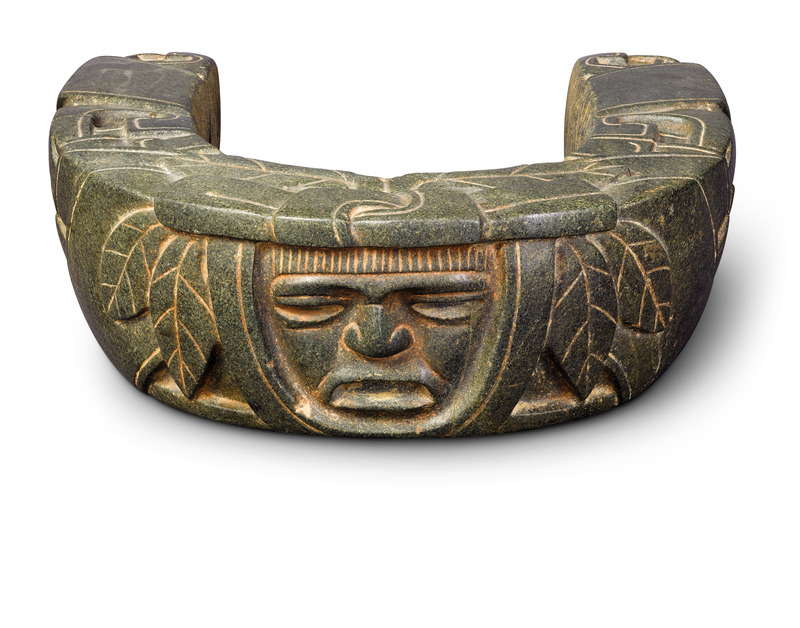This photograph showcases an ancient, semi-circular stone or bronze artifact resembling a horseshoe or half-moon shape, with a flat top surface. The artifact, which might be heavy and solid, sits against a plain white background and radiates a greeny-grey, earthy tone. At the center of the front surface, a face is meticulously carved in relief, featuring prominent eyes, a large nose, and an open mouth. This face is accented with bronze-like highlights enhancing the individual strands of hair, eyebrows, and other facial details. Flanking the face, intricate leaves are carved into the stone, their veins accented with the same bronze-like tint. Additionally, the top of the piece is adorned with swirling patterns and random scribbled lines, while the lower part features triangle carvings. The overall appearance of this artifact suggests it could be an ancient relic or a tribal piece, possibly Mayan, with its weathered yet detailed craftsmanship.